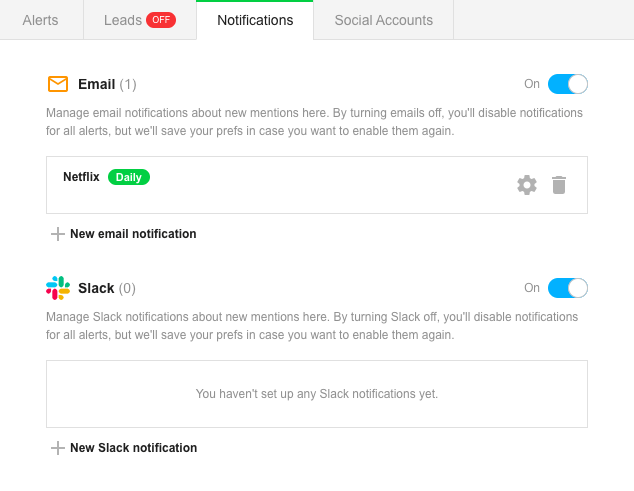The image is a detailed screenshot of a web page dedicated to managing notifications. At the top, a grayish bar contains four tabs: "Alerts," "Leads," a tab with a red notification labeled "Off," and the currently active tab, "Notifications," marked by a thin green line at its top edge. Adjacent to this is the "Social Accounts" tab. The main body of the page has a white background, with a primary section at the top labeled "Email (1)" accompanied by an orange email icon, indicating that email notifications are enabled.

A description underneath this section explains that users can manage email notifications for new mentions and that disabling emails will turn off all alerts, but preferences will be saved for future use. Below, there is a boxed entry for "Netflix" with a "Daily" label in green, flanked by settings and trash icons to the right. Following this box, a plus sign precedes the text "New Email Notification" in black.

Further down, a section for "Slack (0)" is preceded by a Slack icon, showing that Slack notifications are also enabled. The accompanying text outlines that users can manage notifications for new mentions on Slack, with a similar note about preserving preferences if notifications are turned off. The section concludes by stating that no Slack notifications have yet been set up.